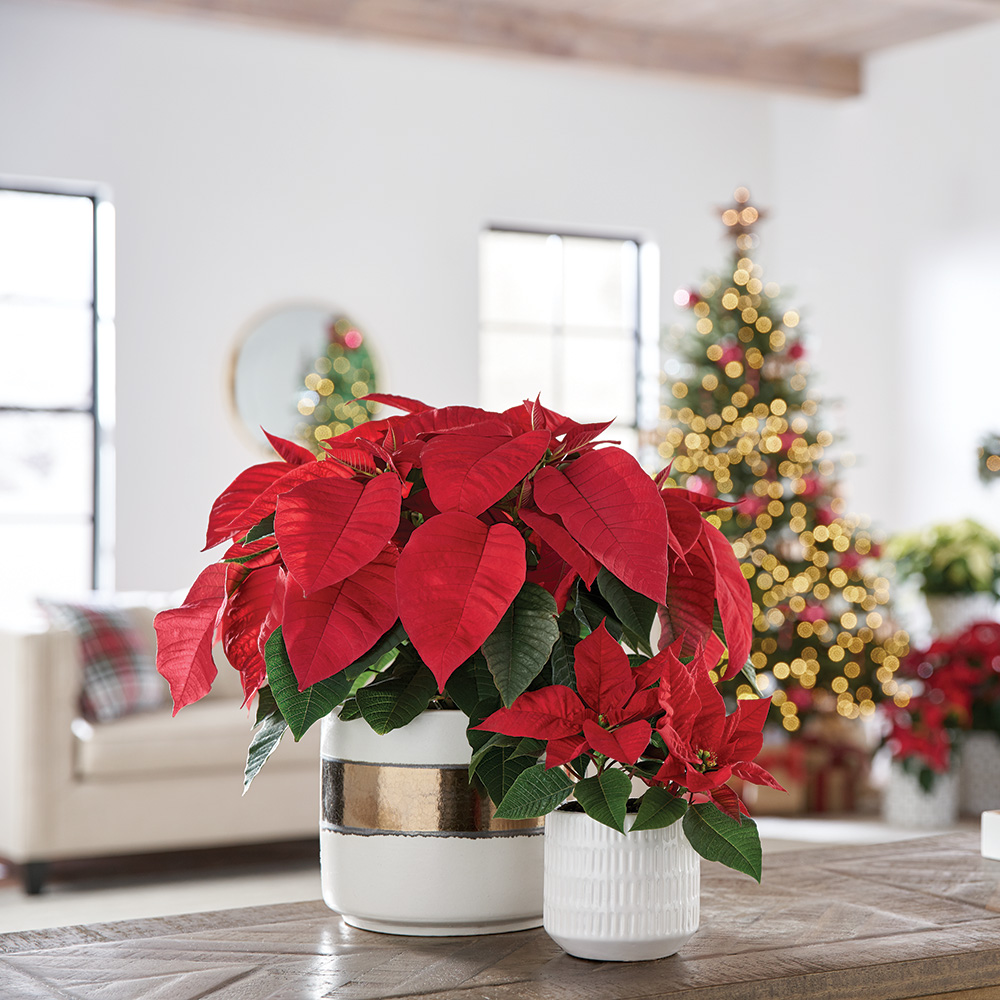In a cozy and festive setting, a close-up captures two vibrant poinsettia plants resting on a stone surface table. The larger poinsettia takes center stage in a white pot adorned with a gold stripe, while the smaller plant, with two blooms, sits just to the right. Both plants are healthy and robust, exhibiting lush red blooms. To the right in the background, a Christmas tree adorned with glowing gold lights and red ornaments casts a warm, blurred bokeh effect. The table with the poinsettias is positioned in front of a cream-colored sofa, complemented by a plaid Christmas-themed pillow, and below a round wall mirror edged in gold, which reflects the Christmas tree. Behind this cozy setup, two large windows framed in white provide a backdrop, adding to the room's airy and bright atmosphere.